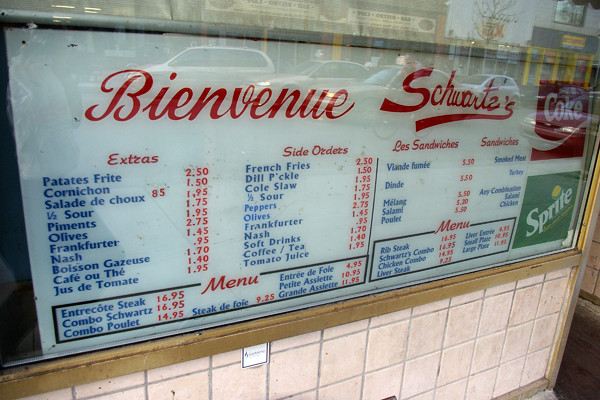In this detailed photograph, a vibrant street scene captures a French menu displayed in the glass window of a quaint walk-up restaurant named "Bienvenue Schwarzes." The name "Schwarzes" stands out in a heavier italic font contrasting the lighter "Bienvenue" above it. The menu is divided into categories including Extras (Extras), Side Orders (Les Accompagnements), and Sandwiches (Les Sandwiches), all meticulously listed with their respective prices.

Beneath the "Extras" section, several items are listed:
- Pâté Frites (French Fries) - $2.50
- Cornichon (Pickle) - $1.50
- Salade de Chou (Cabbage Salad) - $1.95
- Demi-aigres (Half Sour Pickles) - $1.75
- Piments (Peppers) - $1.95
- Olives - $2.75
- Saucisse de Francfort (Frankfurters) - $1.45
- Nash - $1.95
- Bouteille d'Eau (Water Bottle) - $1.70
- Café au Lait - $1.40
- Jus de Tomate (Tomato Juice) - $1.95

Under "Side Orders," the same items are listed with their corresponding prices, this time in English:
- French Fries - $2.50
- Dill Pickle - $1.50
- Coleslaw - $1.95
- Half Sour - $1.75
- Peppers - $1.95
- Olives - $2.75
- Frankfurter - $1.45
- Nash - $1.95
- Soft Drinks - $1.70
- Coffee, Tea - $1.40
- Tomato Juice - $1.95

For "Les Sandwiches," several items are mentioned, although some prices are obscured due to the angle of the photograph:
- Viennese Filet - $5.XX
- Mitande - $5.50
- Mijing - $5.50
- Salami - $5.XX
- Poulet (Chicken) - $5.XX

The "Menu" section offers more comprehensive meals:
- Entrecôte (Ribbed Steak) - $16.95
- Combo Schwartz - $16.95
- Combo Poulet (Chicken Combo) - $14.95
- Entrée de Foie (Liver Entrée) - $4.95
- Petite Assiette (Small Plate) - $10.95
- Grande Assiette (Large Plate) - $11.95
- Steak de Foie (Liver Steak) - $9.25

On the right side, the English translation aligns with the French versions:
- Ribbed Steak - $16.95
- Schwartz Combo - $16.95
- Chicken Combo - $16.95
- Liver Steak - $9.25
- Liver Something - $4.95
- Small Plate - $10.XX
- Large Plate - $1X.XX

Additional elements in the photograph include a Coca-Cola sign, a Sprite sign, and a pink towel below the clear glass window. You can also glimpse the entrance to the restaurant just beyond the sign, which enhances the inviting ambiance of this charming eatery.